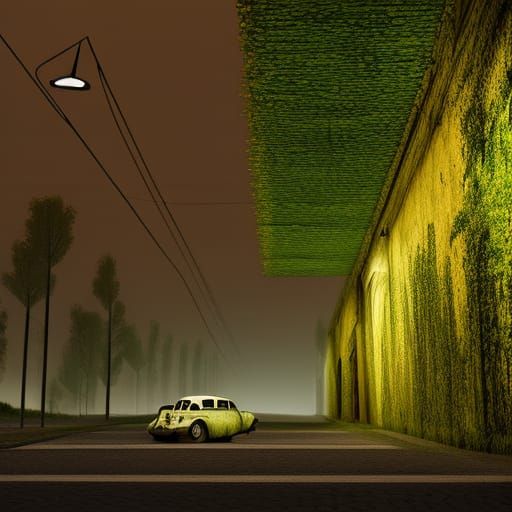The image is a computer-animated artwork resembling a painting with noticeable brush-like strokes. It features a dark, foggy sky in the background. To the left, there are tall, slender trees, resembling palm trees and stick-like trees, which are green in color. At the top left, electric power lines and a hanging white light can be seen. The right side of the image showcases a large stone or concrete wall, heavily covered in green and yellow moss, with a couple of doorways. Portions of green material, possibly roof segments, jut out from the top of the wall, looking like layers of grass. In front of the wall, there is a peculiar, vintage-classical car from the 1940s, 50s, or 60s, with a white top and a light green bottom. The car, which appears to be missing a front tire and has a strange-shaped body and back bumper, is parked in a lot marked with dark green, dark gray, and lighter gray stripes, indicative of parking spaces. The scene is illuminated by the hanging lamp, suggesting an evening time setting.